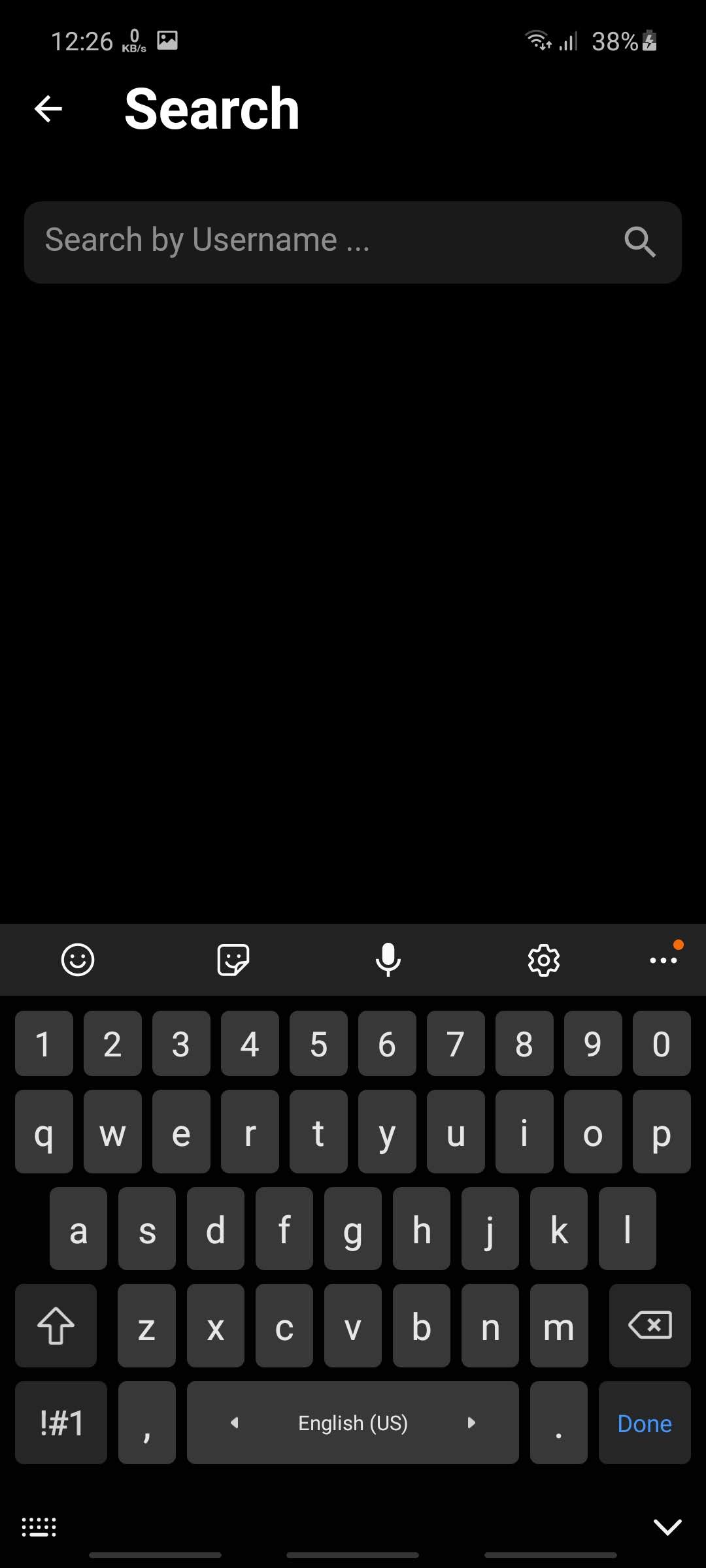A detailed caption for an image showing a screenshot of a phone's search function in dark mode:

---

The screenshot displays the search function on a smartphone operating in dark mode, characterized by a black background. At the upper left corner, the time "12:26" is visible. Adjacent to the time, a symbol representing internet speed shows a value of "0 KB/s." The Instagram logo, indicating attempted access to Instagram, appears beside it. On the upper right-hand corner, icons indicating Wi-Fi signal strength, cell phone signal strength, and a battery level of "38%" are visible, with the phone being plugged into a charger at the time of the screenshot.

Beneath the status icons, there is a white arrow pointing left, followed by the word "Search". Below this, a light gray field with placeholder text "search by username..." is evident, and a magnifying glass icon is placed to the far right. The majority of the screen remains black, representing an empty search field.

At the bottom, a keyboard is displayed. At the top of the keyboard, there are a round smiley face, a square smiley face, a microphone icon, a gear icon, and three dots with an orange indicator above the last gear icon. The full numeric keyboard (1 through 9, and 0) and the QWERTY keyboard are also present in white. In the bottom right corner, the "Done" button is highlighted in blue. The bottom left features a small keyboard icon, accompanied by a down arrow on the right side.

---